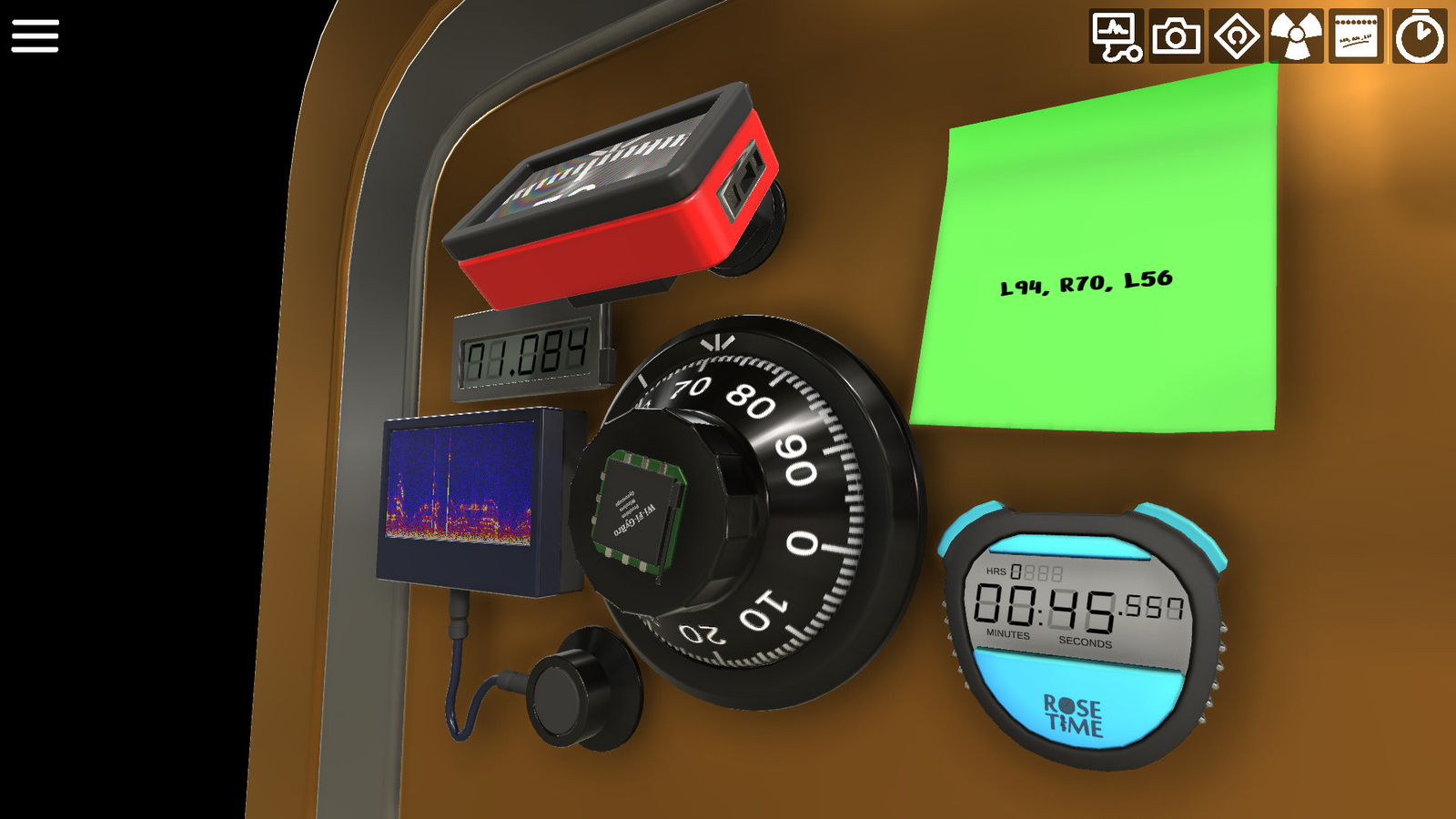The image portrays a complex array of controls and gauges mounted on a goldish-bronze, vertical surface, bordered by a steel-colored edge on the left. The detailed composition features a black combination lock dial, reminiscent of a locker dial, prominently showing white numerals and centered by a computer chip. Adjacent to this, on the right, is a green post-it note displaying the coordinates "L94, R70, L56" in black text. Directly beneath the post-it note is a stopwatch stopped at approximately 45 seconds, labeled "Rose Time". To the left of the lock, a thermal reader connected by a wire to a black module sits below a digital LED meter with a gray outline. Above this meter is a red box with a black rim, possibly another gauge. In the upper left of the image are three vertical white lines against a black background, while the top right corner houses several navigational icons, including a camera symbol, radioactive symbol, and a stopwatch symbol. The entire scene, viewed from an angled perspective, exhibits a stylistic photographic realism, evoking an intricate and somewhat mysterious control panel often seen in video games.